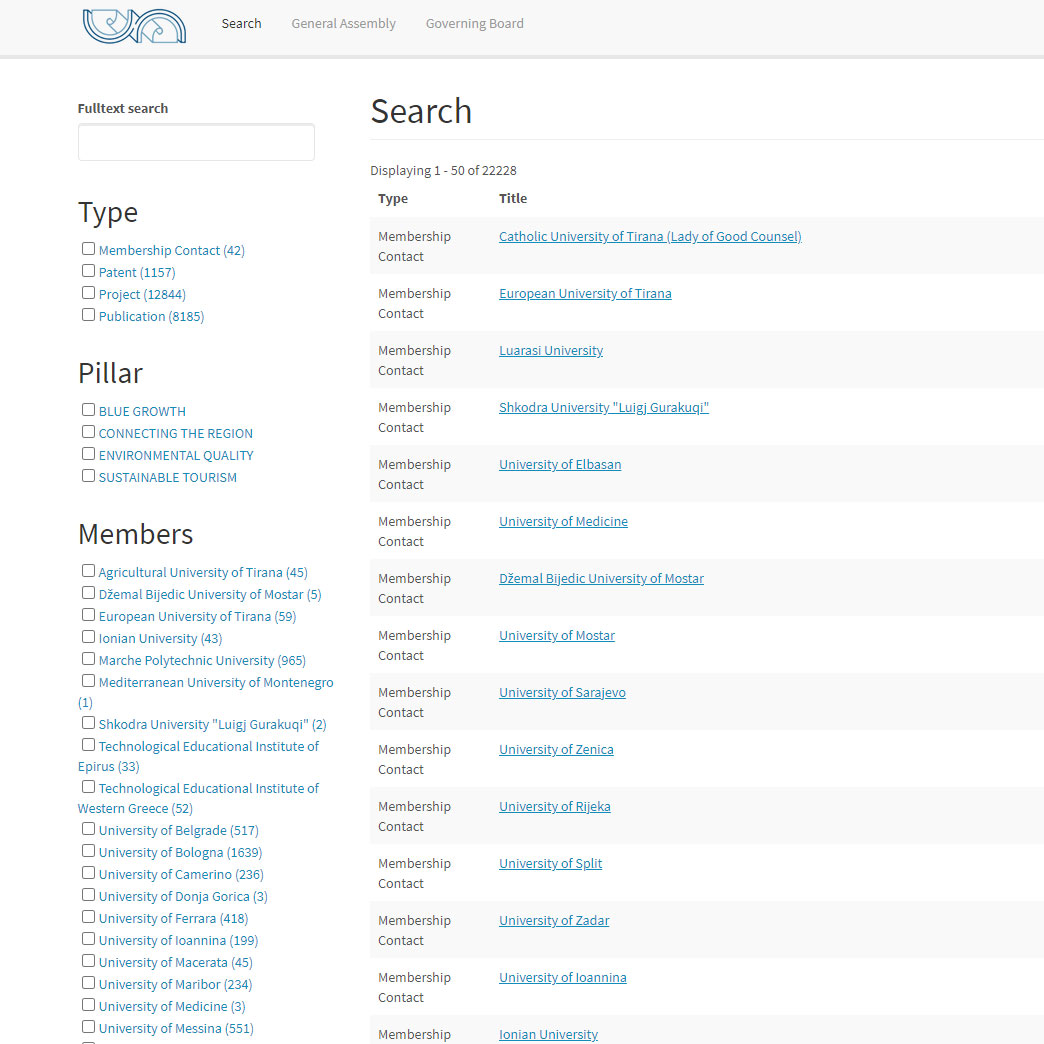The image depicts a screenshot of a website interface. At the very top, there is a header with a logo that is not clearly identifiable, followed by a darker gray search bar. In lighter gray text, "General Assembly" and "Governing Board" are displayed below the search bar.

Beneath the header, the layout is divided into two main columns. The left column includes sections titled "Full Text Search," and below it, "Type," which is followed by categories such as "Membership," "Contact," "Patent," "Project," and "Publication." Further down, another subject section is titled "Pillars," listing "Blue Growth," "Connecting the Region," "Environmental Quality," and "Sustainable Tourism."

The following section, "Members," features a long list of universities and institutes. The first few listed are "Agricultural University of Tirana," "University of Mostar (partially readable: Dezembel Bejidek University of Mostar)," "European University of Tirana," and "Ionian University."

In the right column, a "Search" header is displayed with the information "Displaying 1 to 50 of 122,228." Below this, there are two headings, "Type" and "Title," followed by a list of links to various universities. The first entry is "Membership Contact" with a link to the "Catholic University of Tirana, Our Lady of Good Counsel," accompanied by more links to different universities.